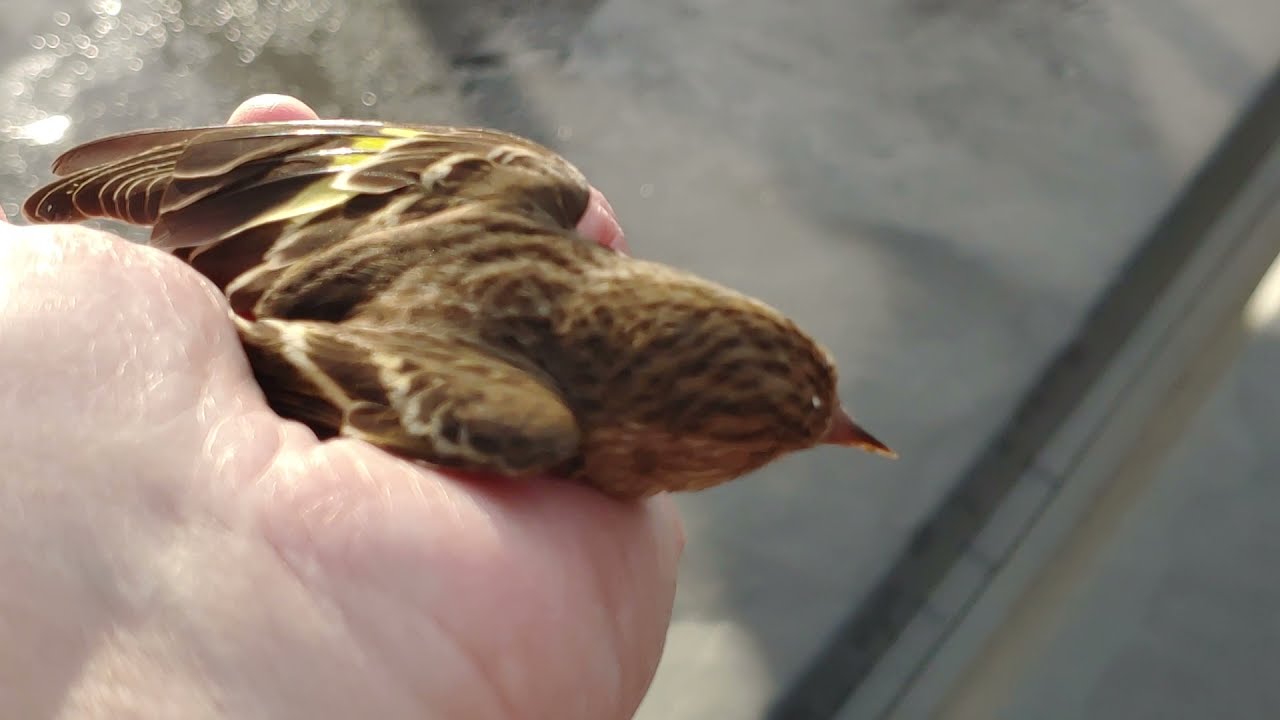The photograph captures a slightly blurred yet focused scene of a small brown bird resting in the palm of a Caucasian person's left hand, viewed from above. The hand is positioned with the palm facing up, revealing numerous wrinkles and lines, with the fingertips peeking up around the bird, suggesting a gentle grip. The bird's head is centrally placed in the image, facing to the right. The bird has a small, pointed beak and its feathers display varying shades of brown with distinctive yellow stripes running through them. Notably, its wings and some inside feathers also exhibit white and yellow hues. The background of the image is a mix of indistinct elements, potentially resembling either water or a glass surface, with patches of white and gray and some shadow effects. The right side of the image is mainly empty, save for a gray line extending horizontally across the bottom, further emphasizing the bird and hand as the focal points. The light is illuminating the scene from the lower left, casting subtle shadows and adding depth to the intricate details of the bird's feathers and the texture of the palm.